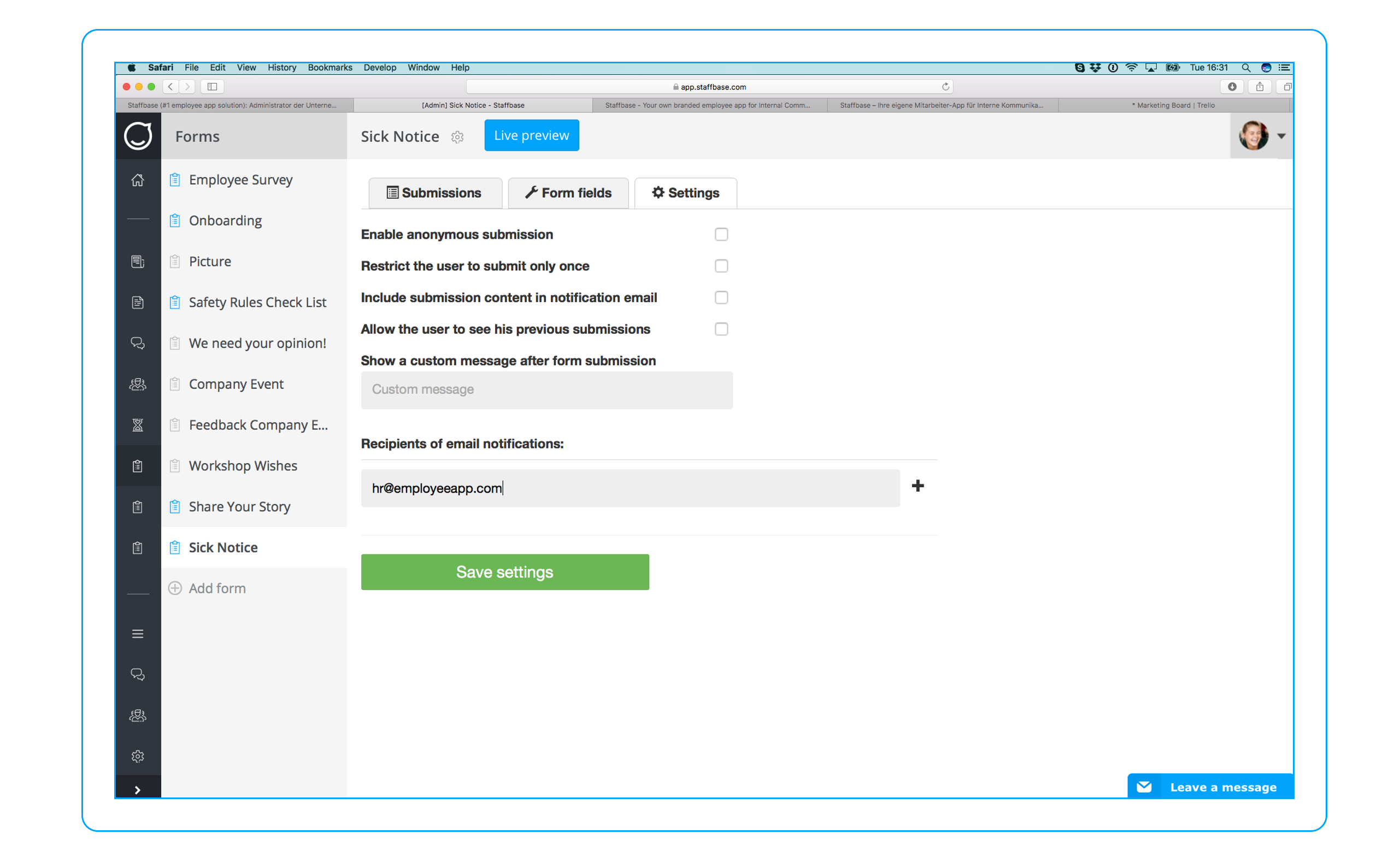Screenshot of a computer interface displaying a form management system. On the far left, there is a vertical black toolbar. Next to it, within a grey box, the following categories are listed: Forms, Employee Survey, Onboarding, Picture, Safety Rules, Checklist, We Need Your Opinion, Company Event, Feedback, Company Workshop, Wishes, Share Your Story, Sick Notice, and Add Form.

To the right of this menu, the focus is on the "Sick Notice" form. At the top, "Sick Notice" is highlighted, and directly below, a blue box labeled "Live Preview" is visible. Beneath this, several sections appear: "Submissions" and "Form Fields," both within grey boxes, followed by "Settings" in a white box. The background of this interface is entirely white.

Within the settings section, several options are listed but unchecked: "Enable anonymous submission," "Restrict the user to submit only once," "Include submission content in notification email," "Allow the user to see his previous submissions," and "Show a custom message after form submission." Below the last option, there's a grey box labeled "Custom Message."

Further down, the recipient of the email notifications is specified as hr@employeeaarpp.com, and there is a green box labeled "Save Settings."

In the bottom right corner of the interface, a blue box titled "Leave a Message" is positioned. In the upper right-hand corner, there is an image of a woman, presumably the owner of the computer.